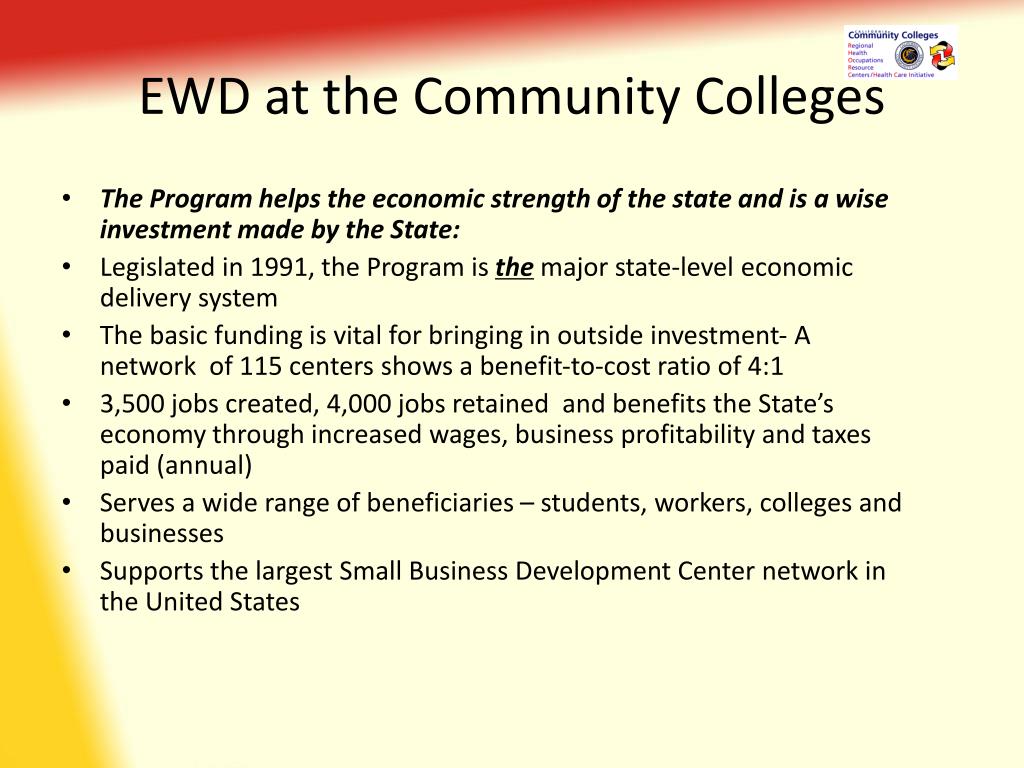The presentation slide is densely packed with information, primarily comprising text. The background is predominantly beige, featuring a red triangular gradient band across the top and a yellow triangular gradient band along the bottom left corner. At the top center, bold black text reads "EWD at the Community Colleges." In the upper right corner, there's a white rectangle containing blue text that says "Community Colleges," accompanied by two logos - one circular and one colorful. 

Below the title, a statement in bold and italicized text emphasizes that the program enhances the state's economic strength and is a wise investment. The slide contains six bullet points detailing various program benefits and features:
1. Legislated in 1991, the program is a major state-level economic delivery system.
2. Basic funding is crucial for attracting outside investment.
3. A network of 115 centers demonstrates a benefit-to-cost ratio of four to one.
4. The program has created 3,500 jobs and retained 4,000 jobs, benefiting the state's economy through increased wages, business profitability, and annual taxes paid.
5. It serves a diverse range of beneficiaries, including students, workers, colleges, and businesses.
6. Supports the largest Small Business Development Center network in the United States.

Overall, the slide communicates the significant impact of the EWD program on the state's economic development.